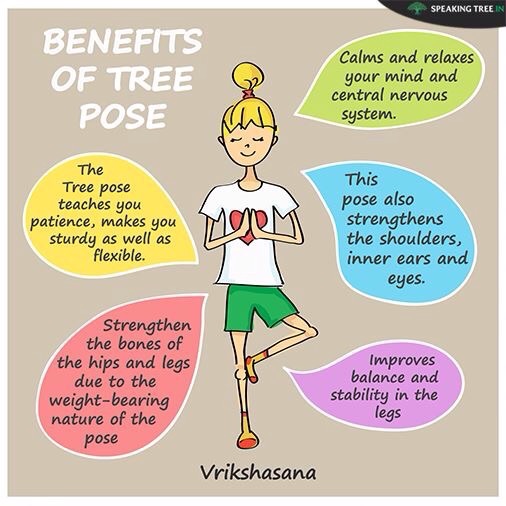The poster features a cartoon character of a thin, blonde girl with a poof on top of her head, wearing a white shirt with a red heart and green shorts. She is standing in a tree pose, smiling, with her hands together. Her socks are yellow and red. The background of the image is light purple. 

On the top left, the title "Benefits of Tree Pose" is written in white letters. Surrounding the girl are five thought bubbles, each shaped like cylindrical leaves, each highlighting the health benefits of the tree pose:
1. The green bubble, located on the top right, states "Calms and relaxes your mind and central nervous system."
2. The blue bubble, below the green one, reads "This pose also strengthens the shoulders, inner ears, and eyes."
3. The purple bubble, directly below the blue one, claims "Improves balance and stability in the legs."
4. The yellow bubble, to the left of the blue and purple bubbles, says "The tree pose teaches you patience, makes you sturdy as well as flexible."
5. The red bubble, at the bottom, declares "Strengthens the bones of the hips and legs due to the weight-bearing nature of the pose."

Overall, the poster is a detailed and colorful illustration highlighting the benefits of practicing the tree pose, with each benefit visually emphasized in distinct, colorful thought bubbles.